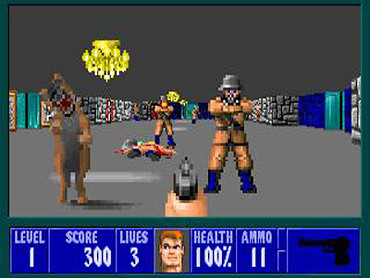Screenshot of a video game in landscape orientation, showcasing a first-person shooter interface. The HUD at the bottom features a blue bar with game stats: Level 1, Score 300, Lives 3, an image of a male character with red hair, Health 100%, Ammo 11, and an icon of a black gun pointed to the left. The game environment depicts three upright targets and one fallen target amidst a maze of gray, blue, and green building blocks and materials. A yellow chandelier hangs in the upper left corner. The background gradient transitions from dark gray at the top to light gray at the base, adding depth to the setting.